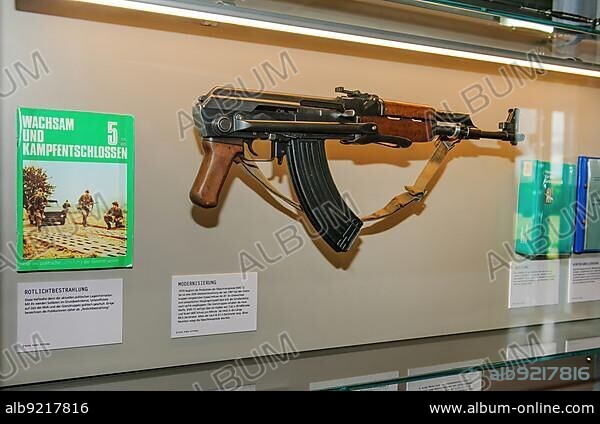This detailed photograph captures a Kalashnikov-style rifle, prominently displayed within a glass display case, likely situated in a museum. The rifle, elongated and showcasing vintage features, includes a polished wooden grip, a banana clip, and a forward wooden hand handle, all of which are immaculately shiny. The thin, dark blue barrel extends outward, culminating in a sight at the very end. A distinctive olive drab strap is affixed from the butt of the weapon towards the front muzzle. 

Positioned on a solid gray board, the rifle is flanked by illustrative depictions, possibly of historical soldiers wielding similar firearms, and accompanied by descriptive text, which appears to be in a foreign language, possibly German. The display case also carries a prominent watermark with the text "ALBUM" stretching across the image, and a website, www.album-online.com, is visible in the bottom right corner. The reference "ALB 9217816" is noted on the lower left-hand side, adding to the specificity of the documentation.

Overall, the image, reflective due to its glass enclosure, suggests a historical context, potentially showcasing a weapon from past conflicts, further enforcing its authenticity and significance as a museum exhibit.